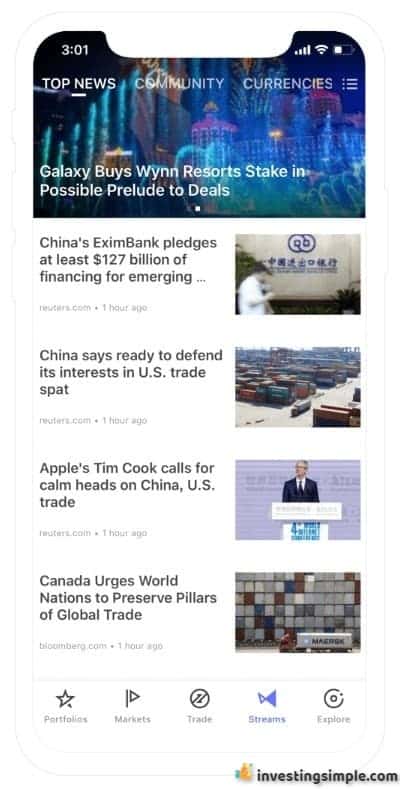This detailed caption provides a comprehensive description of a screenshot showing a news webpage:

"The screenshot depicts a news webpage featuring a navigation menu at the top with three buttons labeled 'Top News,' 'Community,' and 'Currencies.' To the right of these buttons, there is a white menu icon. The 'Top News' button is underlined in white, indicating the current section being viewed. Below the navigation menu is a prominent image of a casino with a headline underneath that reads, 'Galaxy Buys Wind Resort Stake in Possible Prelude to Deals.'

Beneath this headline, there are four article previews listed vertically. Each preview consists of a headline on the left and a thumbnail image on the right. 

1. The first article is titled 'China's Ex-Im Bank Pledges at Least $127 Billion of Financing for Emerging...' with a news source attribution to Reuters.
2. The second article headline reads 'China Ready to Defend Its Interests in U.S. Trade Bets,' though the news source is not mentioned.
3. The third article and its details were not described in the voice caption.
4. The fourth article's source is identified as Bloomberg.com, but the headline was not articulated.

The design and layout provide a structured and informative view, ensuring users have easy access to the latest news and updates."